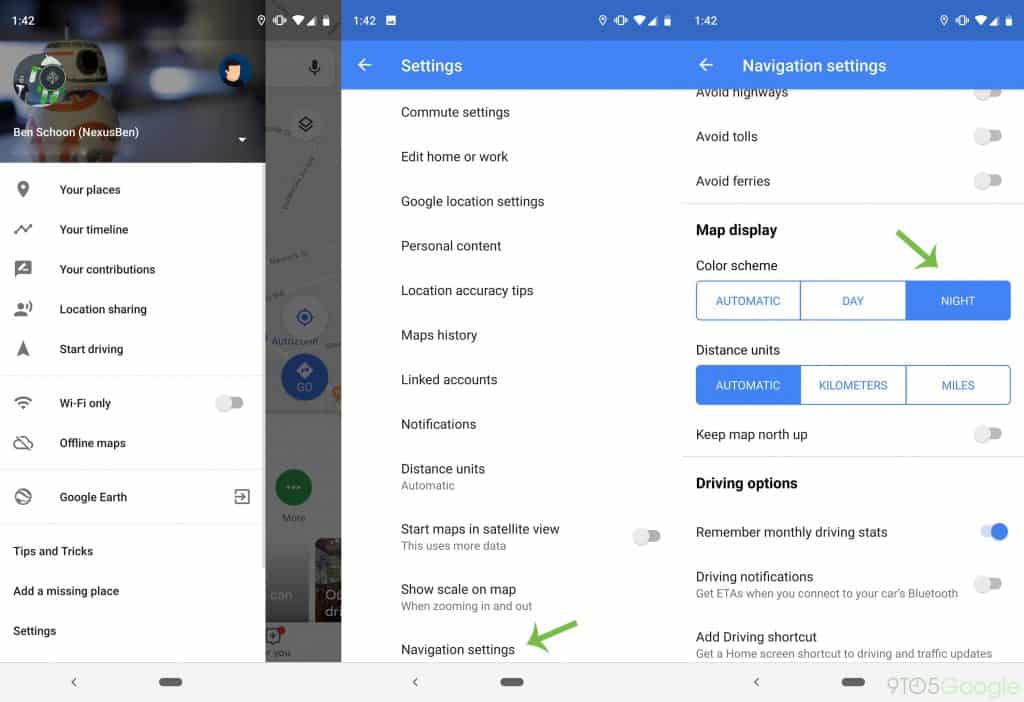The left side of the image features a sheer gray bar that partially reveals a picture underneath, extending further. Alongside the sheer gray bar are several numbers. Below this section, there is an image highlighting a gray circle containing a robot illustration with white text underneath. Adjacent to the gray circle is a blue circle with the outline of a man's face, lacking detailed features such as eyes, nose, and mouth.

Beside this setup lies a sheer gray rectangle running vertically from top to bottom. At the top of this rectangle, a series of symbols are visible, including a Wi-Fi symbol and a battery icon, accompanied by more numerical data mentioned within a blue rectangle. The rectangle contains not only a white square filled with blue elements but also repeats several of the initial symbols and numbers, extending to a similar layout on the far right.

The left column further features a series of icons and text labels, namely:
- A map symbol labeled "Your Places".
- A diagram symbol labeled "Your Timeline".
- A speech bubble marked "Your Contributions".
- A person icon with two curved lines labeled "Location Sharing".
- An upwards-pointing triangle labeled "Start Driving".
- A Wi-Fi icon labeled "Wi-Fi Only".
- A cloud symbol with a line through it labeled "Offline Maps".
- A circle with lines labeled "Google Earth".
Additionally, options for "Tips and Tricks", "Add a Missing Place", and "Settings" are listed.

To the right side of the screen is a lighter blue rectangle positioned beneath a darker blue one. This area comprises:
- Leftward-pointing arrows, one labeled "Settings" and another "Navigation Settings".
Below the "Settings" label, a list of twelve items descends, marked by a green arrow on the twelfth item. More text appears to the right, separated by a gray line. Adjacent to this text is a light gray circle and a darker gray bar, alongside the text "Map Display". Underneath this section:
- "Color Scheme" with options in blue outlined rectangles: "Automatic", "Day", and a filled blue rectangle indicating "Night," with another green arrow pointing at the blue rectangle.
- Options for "Distance Units" with choices in blue-outlined rectangles: "Automatic", "Kilometers", and "Miles".
- "Keep Map North Up", with accompanying gray circles and bars.
- "Driving Options" including "Remember Monthly Driving Stats", "Driving Notifications", mentioned on a light blue bar with a darker blue circle and additional text underneath.

Further down, another light gray bar repeats the structure of leftward-pointing arrows, concluding with the label "9T05 Google".